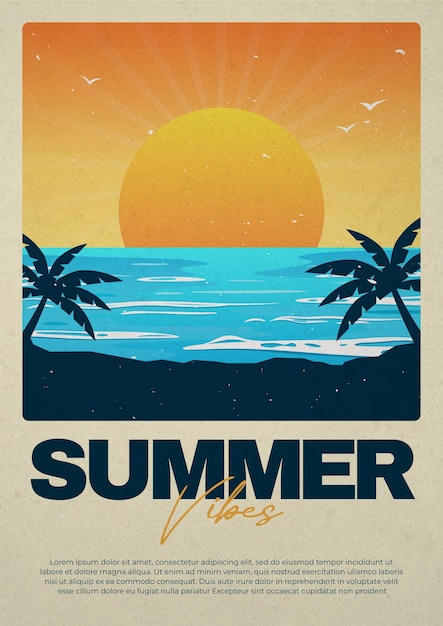This poster features an evocative beach scene set against a beige background. Dominating the composition is a stylized, vibrant illustration, rather than a photograph. A massive, bright orange sun is partially setting into calm, turquoise blue waters, its rays radiating through an orange-yellow gradient sky. The water is adorned with artistic white wave designs. The shore is depicted with striking black sand, framed on either side by dark silhouettes of palm trees.

In the sky, several basic white bird drawings are scattered, with three being prominently larger. Below the image, the phrase "Summer Vibes" is displayed; "Summer" is written in large navy blue block letters, and "vibes" in a smaller, golden handwritten style. The bottom of the poster features four lines of small, unreadable text in what appears to be lorem ipsum, adding a touch of design. 

This artistic representation captures the essence of a tranquil, tropical sunset with bold, contrasting colors and simple, clean illustrations.